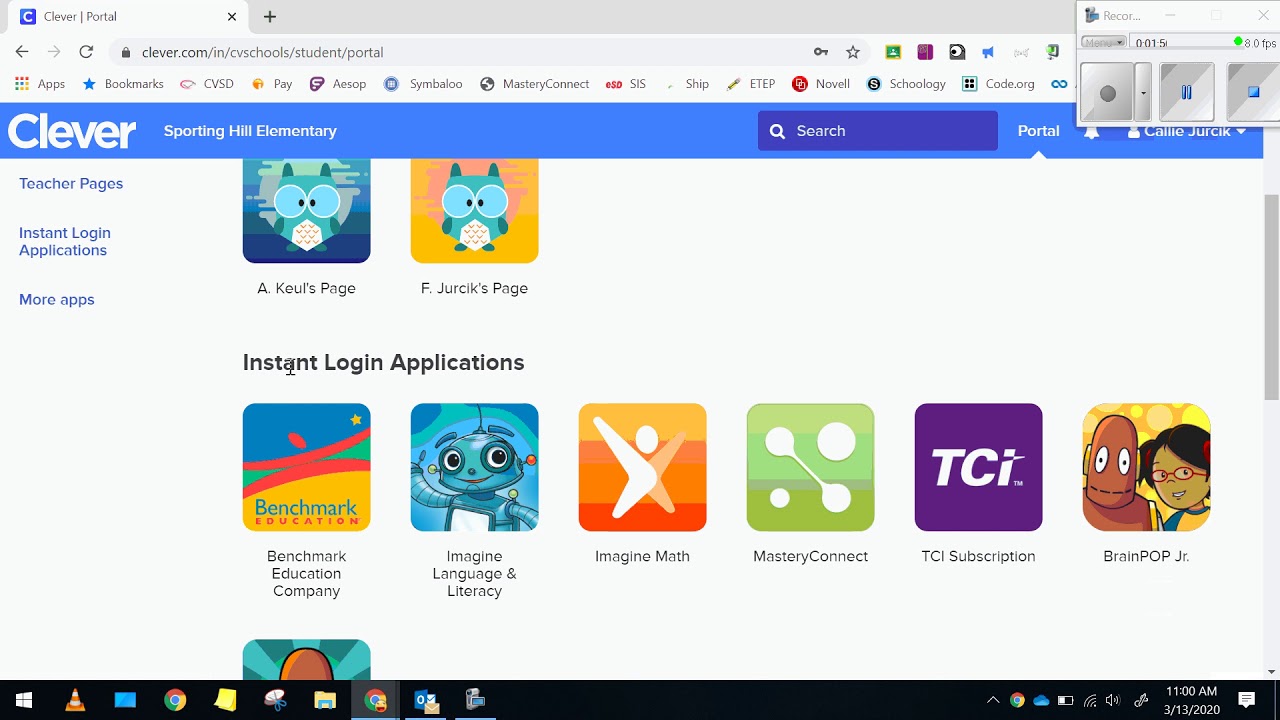This image is a screenshot from a website displayed in portrait mode. In the upper right-hand corner, there is a pop-up screen with "RECOR" displayed, and underneath it, a small text reads "0.01." Adjacent to this text is a small gray-green dot indicating "8.0 FPS." Below this, there are several controls, including a stop button and a pause button rendered in blue, with an option to close the pop-up.

In the main screen, the upper left-hand corner shows the "CLEVER portal." Directly underneath, the URL "clever.com/in/cvschools/students/portal" is visible. Below the URL are various app bookmarks: "CVSD pay," "ASAP," "Symbaloo," "Mastery Connect," "SIS," "eTEP," "Novels," "Schoology," "Code.org," among others.

The following section, with a light blue background, reads "Clever Sporting Hill Academy," followed by a blue search bar with the label "Portal." This page appears to be the current view. Hidden underneath the pop-up menu, we can slightly see a user profile labeled "Kali J" with "CUK's" nearby. The left sidebar displays options such as "Teacher Pages," "Instant Login Applications," and more app categories. The right column features entries including "A Cool's Page," "F Jurisdic's Page," and others related to instant login applications, occupying the first two rows.